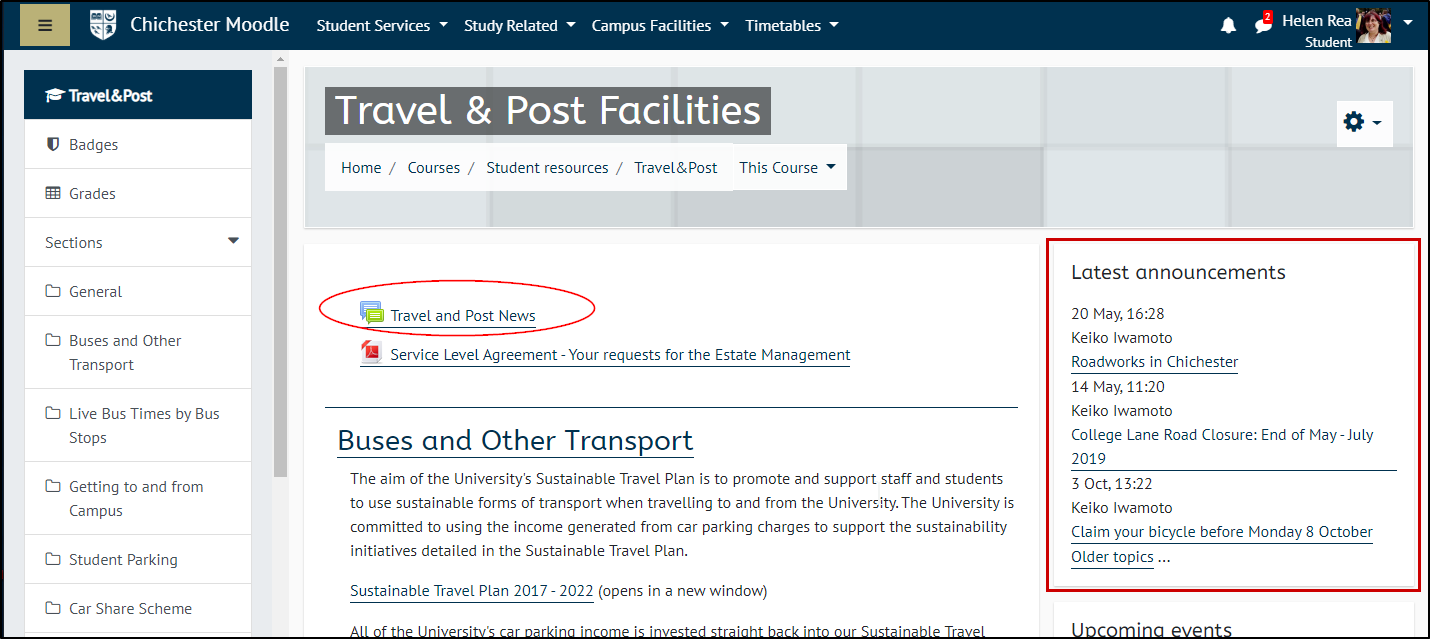The image features a comprehensive and structured layout primarily composed of several distinct sections and visual elements. At the top of the image, there is a long horizontal blue bar. On the left side of this bar, there is a beige-colored square with three small black lines inside. 

To the right of the beige square, white text reads "Chichester Moodle Student Services," followed by categories such as "Study Related," "Campus Facilities," and "Timetables." At the far right end of the blue bar, there is a white speech bubble icon containing a small red circle with the number two inscribed inside it. 

Next to this icon, the name "Helen Ray" is displayed, accompanied by an image of a smiling woman with brown hair. Beneath her name, the text "Student" appears, followed by the phrase "Travel and Post Facilities" inside a gray rectangular box.

Approximately three inches below this, there is a red-circled text that reads "Travel and Past News." To the right of this red circle, a red-outlined square contains the heading "Latest Announcements," followed by the date "20th May 16:28." Below this, there is an underlined announcement stating "College Lane Road Closure End of May-July 2019."

Finally, in the lower right corner beneath this red-outlined square, the words "Upcoming Events" are clearly visible.